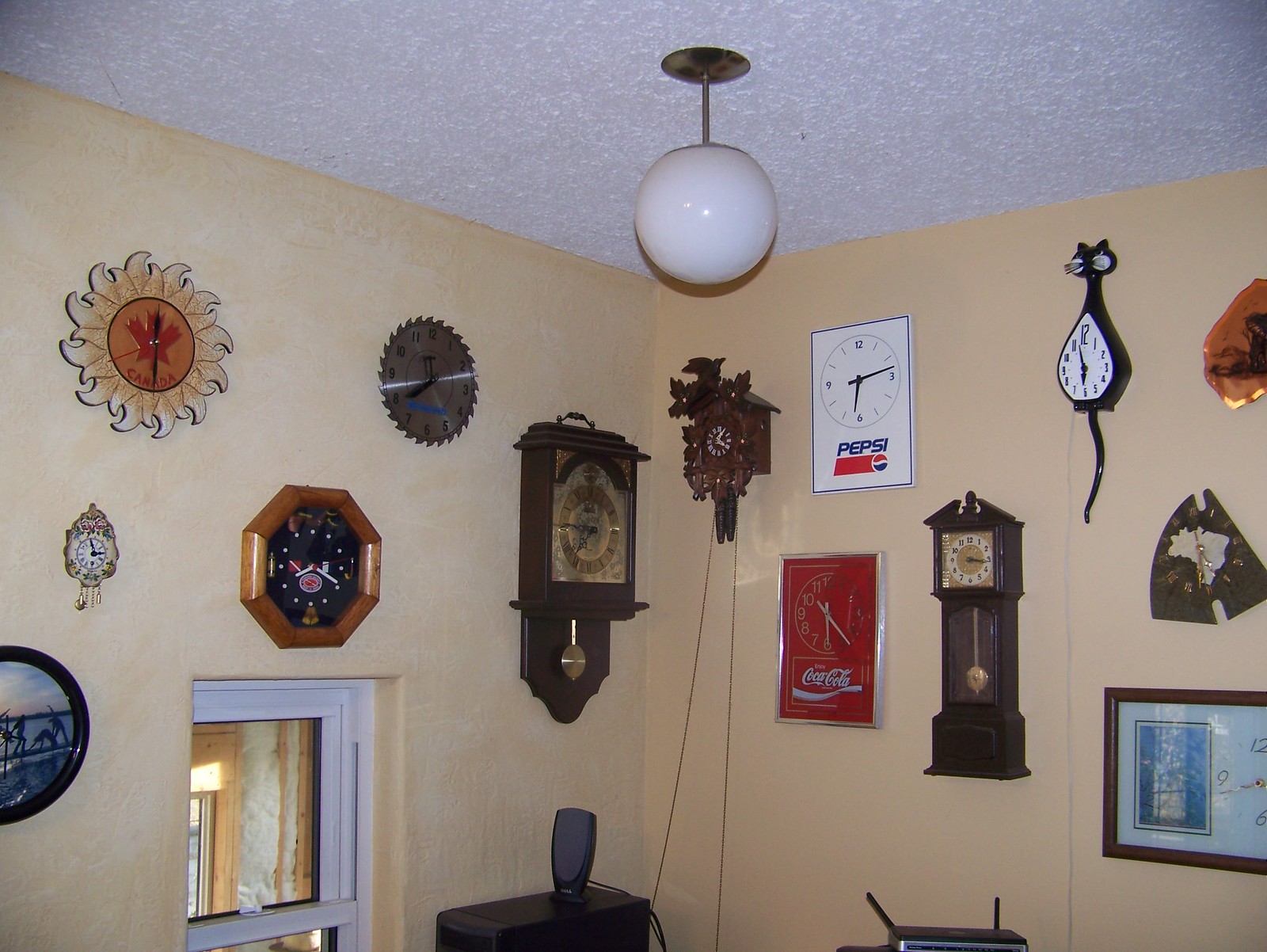The image portrays an eclectic and eccentric room with walls covered in a variety of analog clocks. The walls are a peach or beige color, contrasting with the white, textured ceiling. A distinctive globe lamp with a golden base and a white sphere hangs from the ceiling. The assortment of clocks includes everything from small grandfather clocks to cuckoo clocks, a Coca-Cola clock, a Pepsi clock, an old-school cat clock with a swinging tail, a clock with a Canadian maple leaf, and one made from a circular saw. Additionally, a framed picture in a brown frame and a small desk holding outdated computer speakers and a computer tower occupy the bottom center of the image. The photograph appears to have been taken 10-20 years ago, evident from the quality and state of the technology depicted.